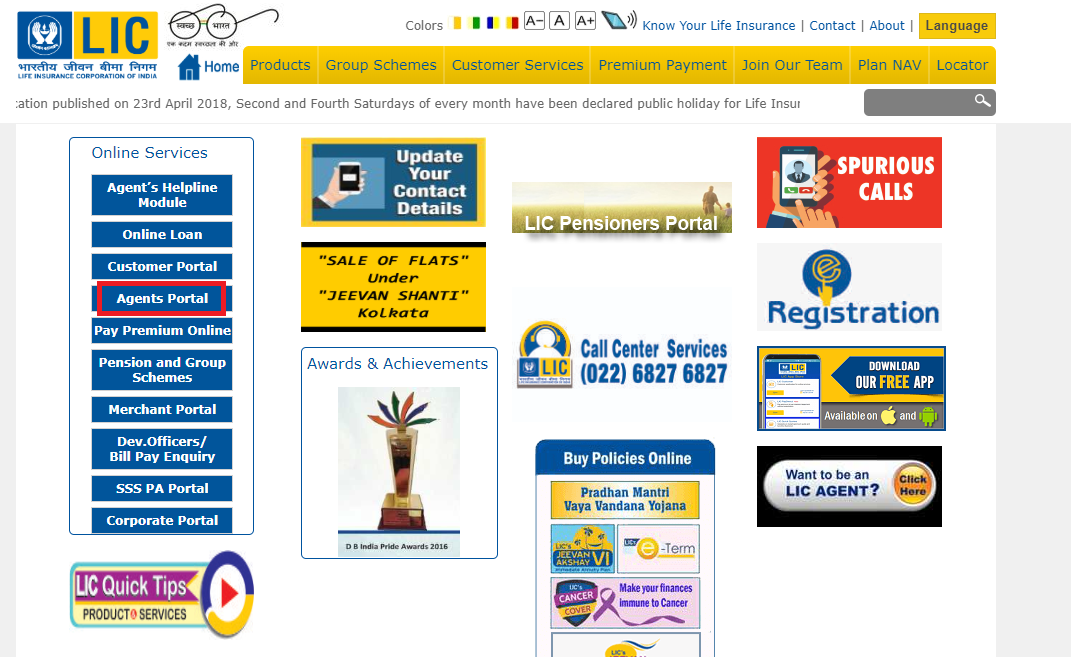**Detailed Caption:**

The image depicts the official website of the Life Insurance Corporation of India (LIC). The homepage features a prominent navigation bar at the top, adorned in yellow with blue text. The navigation options include 'Home', 'Products', 'Groups', 'Schemes', 'Customer Services', 'Premium Payment', 'Join Our Team', 'Plan', 'NAV', and 'Locator'. Adjacent to these, a yellow button labeled 'Languages' is situated, followed by links to 'About', 'Contact', and 'Know Your Life Insurance'.

On the left side of the homepage, there's a vertically aligned navigation pane. This section is filled with blue buttons featuring white text and includes categories for 'Online Services', 'Agent Helpline Module', 'Online Loan', 'Customer Portal', 'Agent Portal', 'Pay Premium Online', 'Pension and Group Schemes', 'Merchant Portal', 'Dev Officers', 'Bill Pay Inquiry', 'SSPA Portal', and 'Corporate Portal'.

The 'Agent Portal' button is highlighted with a red rectangular border. Below the navigation pane, additional information is provided such as 'Update Your Contact Details', 'Sales of Flats under Jeevan Sati Kolkata', 'Awards and Achievements', 'LIC Pensioners Portal', and 'Call Center Services'. Contact information is provided with a helpline number: 022-6827-6827. Further options include 'Buy Policies Online', 'Spurious Calls' with 'S-P-U-R-I-O-U-S' specifically highlighted, 'Registration', 'Download Our Free App', 'Want to be an Agent', and 'An LIC Agent'. This well-structured layout ensures ease of navigation and accessibility for users seeking various services and information.